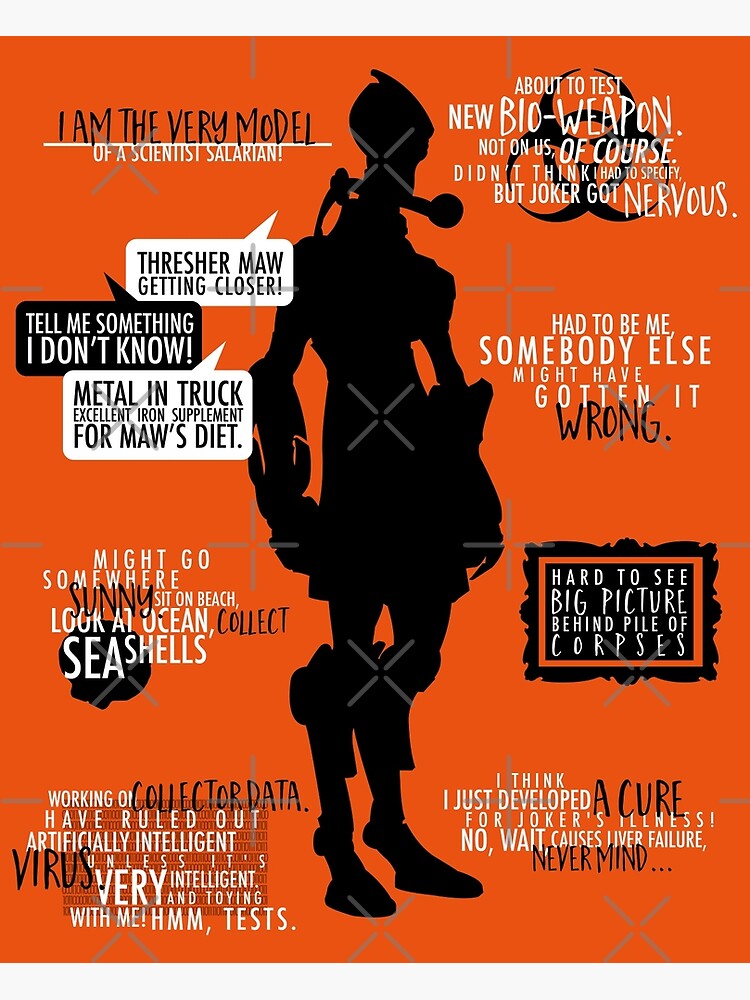The image depicts a large, vertically-oriented graphic set against an orange background, featuring a silhouette of a figure standing in the center. This figure is entirely black, making any specific details indistinguishable, but it's clear that they are clad in armor with cloven feet and a skeleton-like head. A microphone extends from their head or neck region. Overlaying the image are Xs, plus signs, and letters arranged as if seen through a viewfinder, with various text fragments scattered throughout.

The text includes: "I am the very model of a scientist salarian. Thresher Ma getting closer. Tell me something I don't know. Metal in truck. Excellent iron supplement for Ma's diet. Hard to see big picture behind pile of corpses. I think I just developed for Joker's illness. No weight causes liver failure. Never mind. Had to be me. Somebody else might have gotten it wrong. About to test new bioweapon. Not on us, of course. Didn't think I had to specify but Joker got nervous." 

The right side of the image repeats some of these phrases, adding to the chaotic and mysterious atmosphere of the scene. The entire graphic is watermarked.